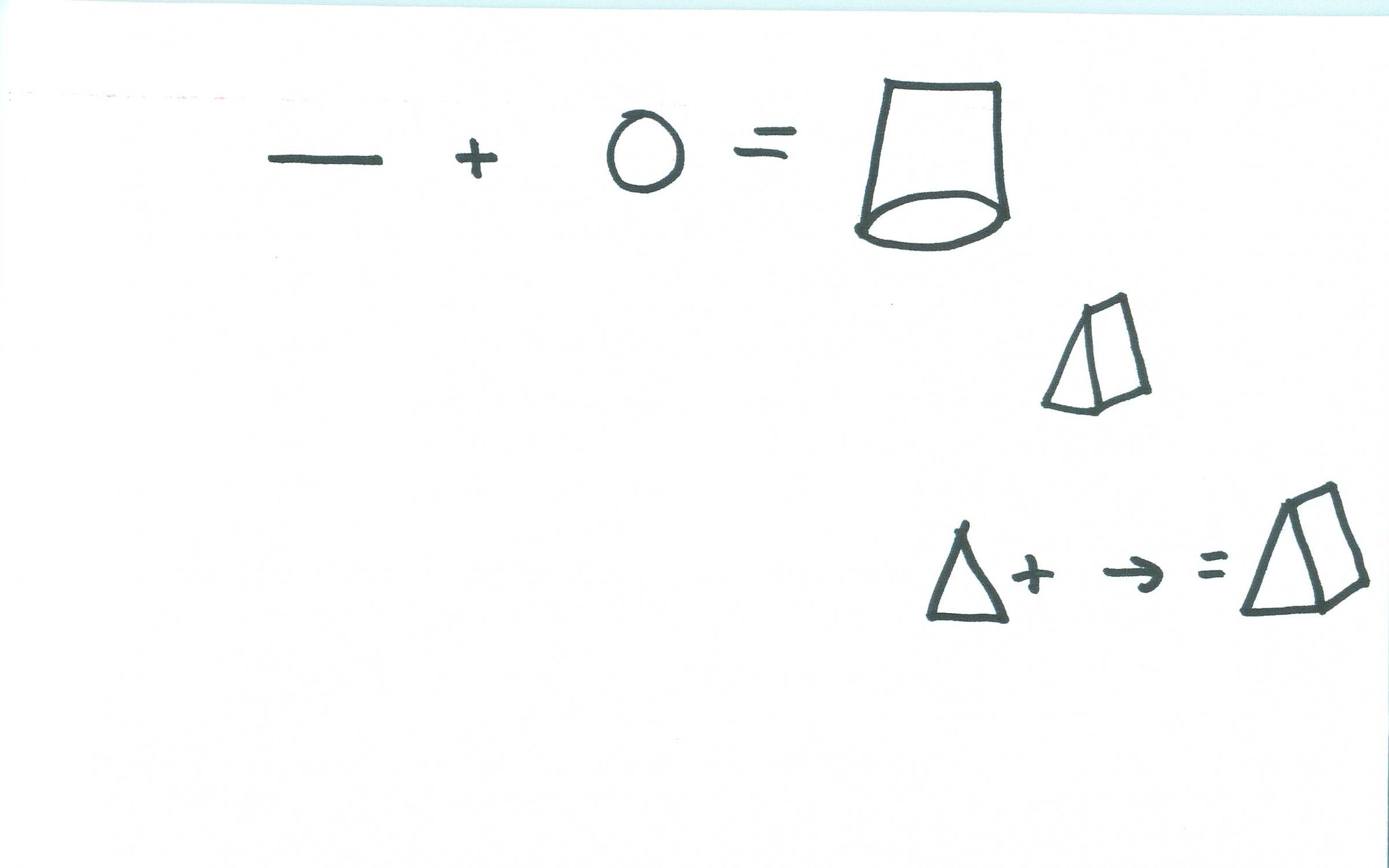The image appears to be a schematic drawing or diagram with specific geometric symbols and annotations. At the top of the image, there is a horizontally dashed line accompanied by a small plus sign and the numeral zero. To the left of this line, there is an equal sign where the upper line is very short compared to the much longer bottom line. Below this level, there is a distinct symbol resembling a square with a circle attached underneath, resembling an overturned wastebasket.

Continuing downward and to the right of this symbol, there is a three-dimensional triangle. This triangle has a short base and elongated sides, with another square attached to its right side. Moving further down and slightly to the left, another triangle is depicted, overlapping slightly on both sides of its top edge. Following this, there is a plus sign, an arrow pointing to the right, and another equal sign. Lastly, one more of the three-dimensional triangles with an attached square is located at the bottom of the image.